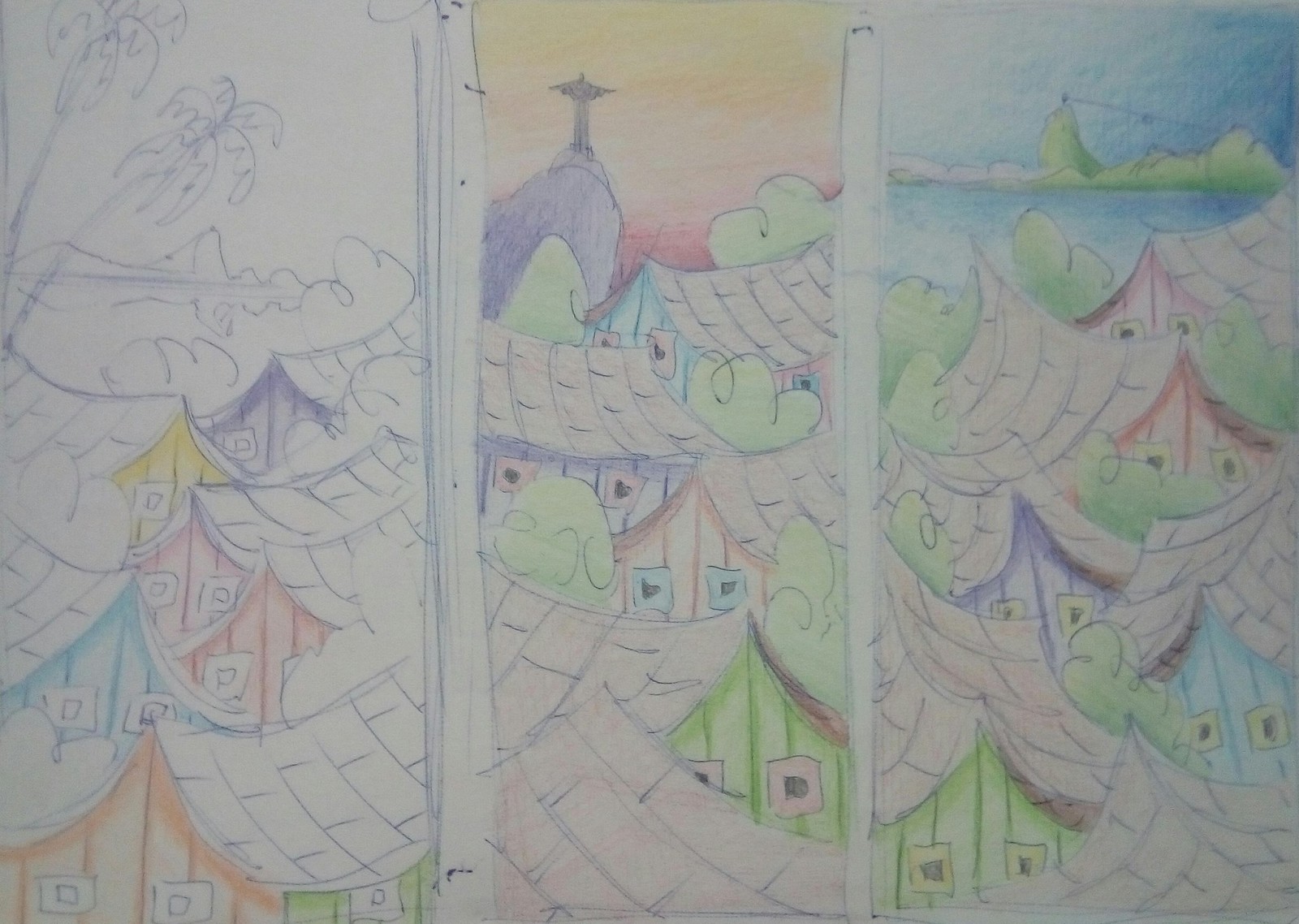This colored pencil drawing is divided into three vertical panels, each separated by long white rectangular lines. The left panel features a cluster of closely packed, colorful houses with vibrant facades in shades of blue, yellow, pink, orange, light blue, purple, and lime green. These buildings, characterized by their whimsical curved A-frame roofs, sit against a backdrop of uncolored pencil-drawn palm trees swaying as if blown by the wind, ocean waves, and distant mountains. 

The middle panel highlights a giant mountain crowned by the iconic Christ the Redeemer statue. The sky here is a striking blend of orange and red hues, giving an impression of a dramatic sunset. Below the statue, the familiar houses reappear with the same vivid colors, accompanied by simplified trees with three-looped foliage. 

The right panel offers a blue lake extending into the background, with softly undulating hills beyond. The sky is distinctly blue, contrasting with the middle panel's fiery tones. The same vibrant, multi-colored houses populate the foreground, interspersed with green tree foliage and shrubbery. In the far distance, a green hill with a tiny depiction of the Christ the Redeemer statue is visible, echoing the central panel's landscape.